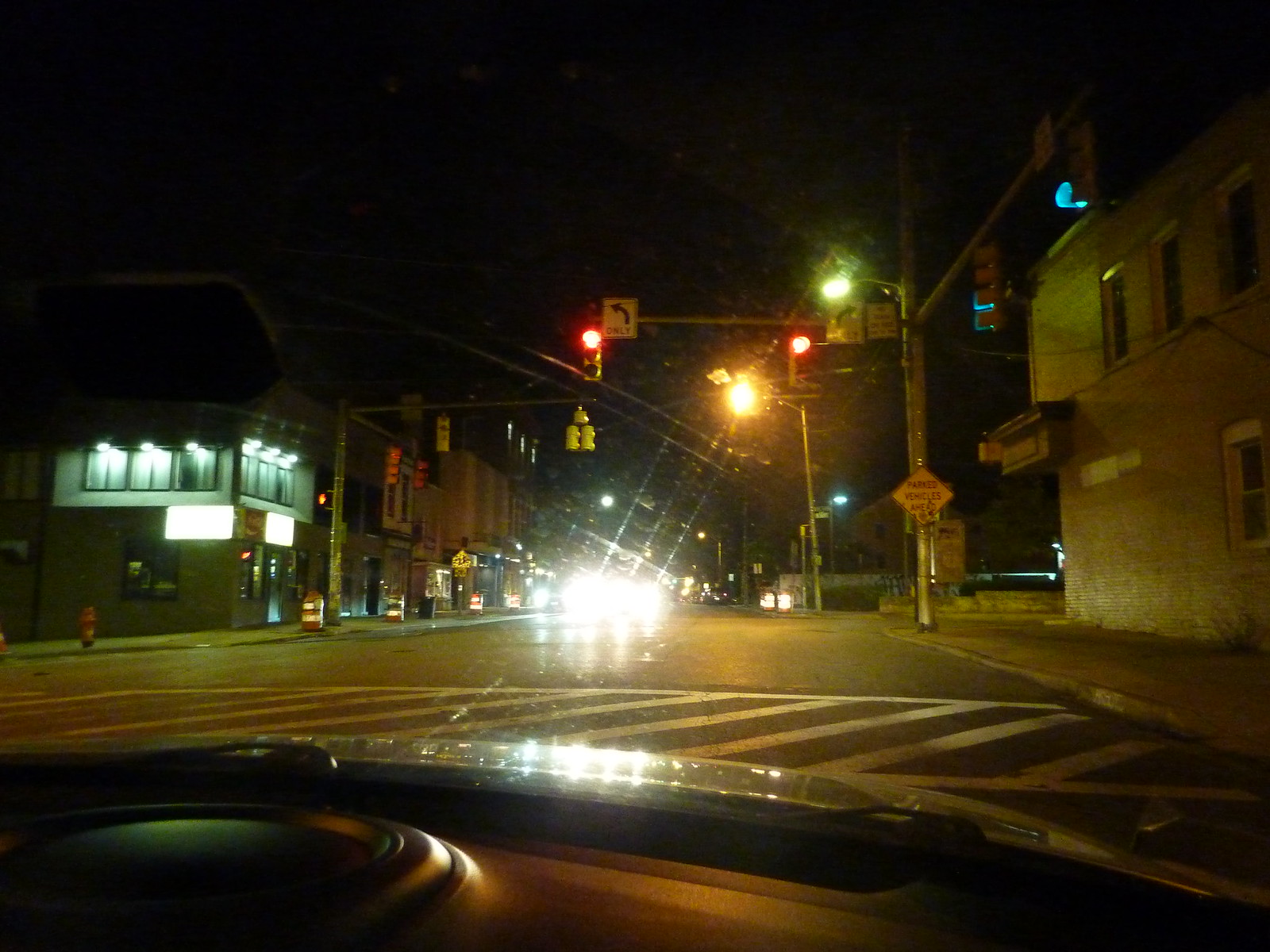A nighttime photograph captures the interior view from within a passenger vehicle, possibly a car, truck, or SUV, halted at an intersection. The dashboard is subtly illuminated by the overhead and front lights, casting a soft glow to reveal its dark color. The hood of the vehicle reflects the headlights from cars ahead, emphasizing the stillness of the scene. The vehicle is positioned just before a marked crosswalk, delineated by bold white lines stretching across the street. Above, a traffic signal mounted on a steel tubular armature towers over the intersection, displaying bright red lights. Attached to the arm are directional signs with arrows pointing left and right. Opposite this vehicle, other cars face towards the intersection, flanked by buildings on either side, all contributing to the serene yet vibrant tableau of a typical urban night.